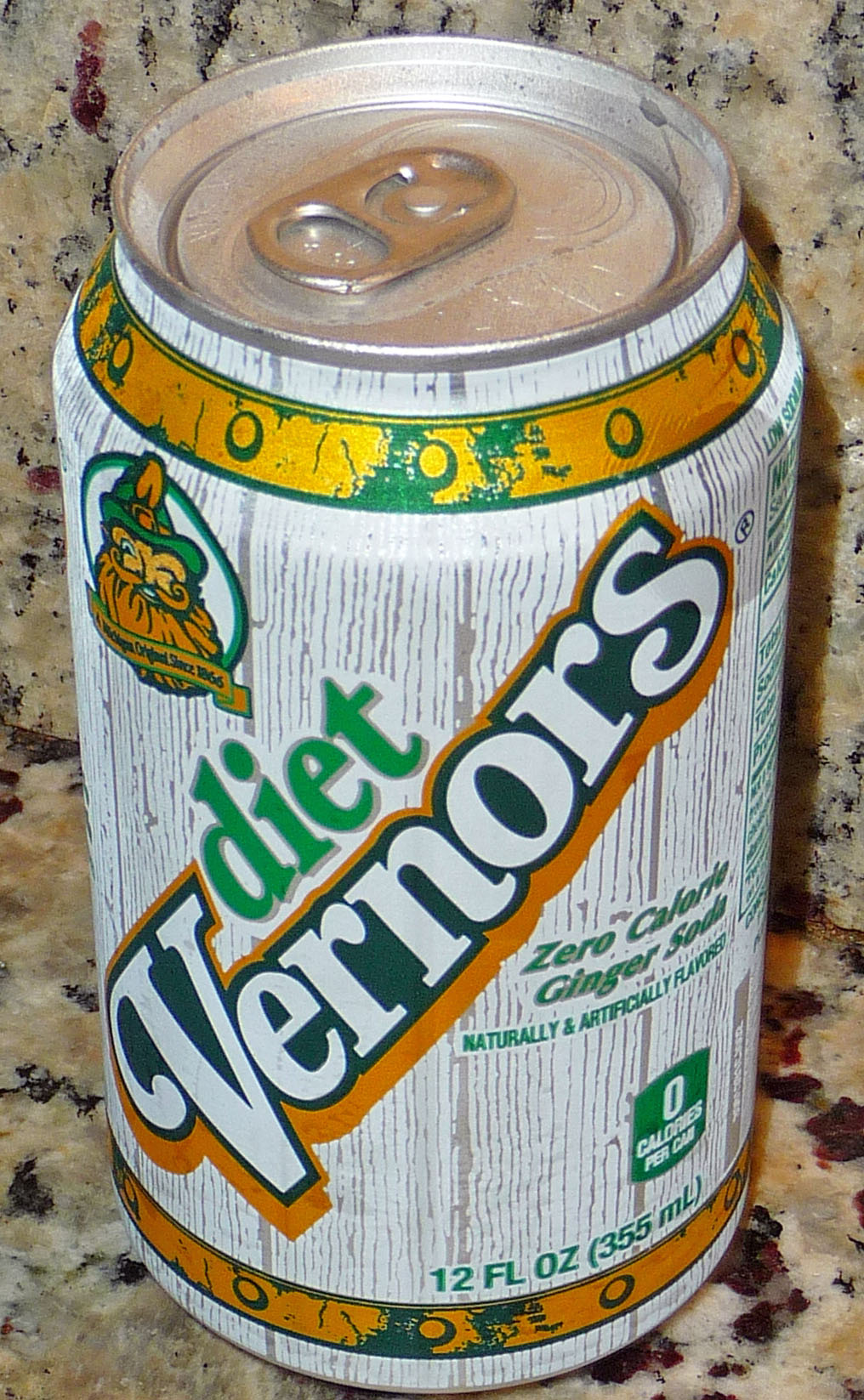**Caption:**

A white, gray, orange, and green Diet Vernors soda can is prominently placed on a marbleized counter featuring an array of red, cream, dark brown, and black hues. The counter's stone-like appearance provides a contrasting and somewhat unattractive background to the can, which is both naturally and artificially ginger-flavored. The front of the can displays the text "Diet Vernors" in bold letters, beneath which it highlights "zero calorie ginger soda, naturally and artificially flavored" and "zero calories per can" in a small green square. The volume of the can is noted as 12 fluid ounces. Both the top and bottom edges of the can are adorned with an orange border featuring intricate green designs.